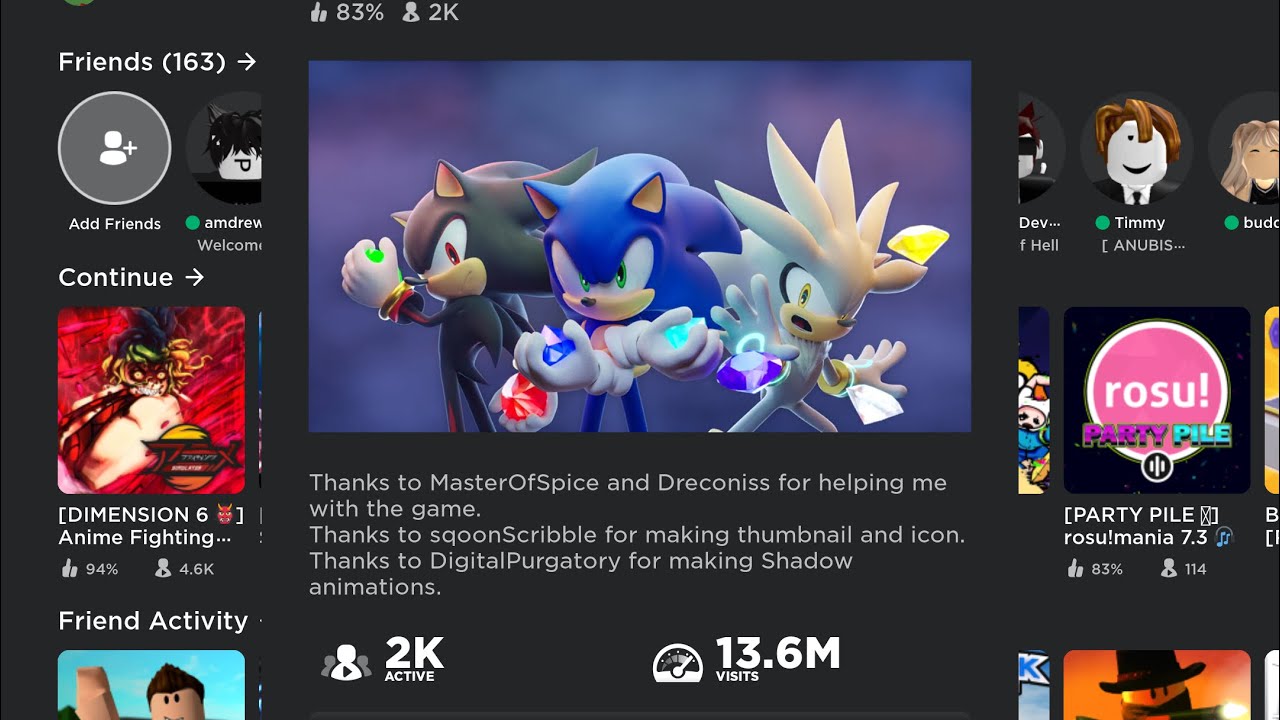This detailed image features a lively computer screen filled with various elements. Along the top, the screen displays "Friends 163" followed by options to "Add Friends." Additionally, there is a section titled "Dimension 6 Fighting" and "Friend Activity."

The lower portion of the image is adorned with several messages of gratitude. It reads, "Thanks to Master of Spice and Draconis for helping me with the game. Thanks to Skwoon Scribble for making the thumbnail and icon. Thanks to Digital Purgatory for creating the shadow animations." 

The image also indicates, "2K active" users and "13.6 million visits."

The middle of the screen showcases characters reminiscent of those from the Sonic comic series. One character, distinctively white, is surrounded by floating petals. Beside it are two cat-like characters — a mischievous blue cat and a brown cat.

Above all these elements is a "Rozu Party Pile" section, creating an overall cluttered and chaotic yet vividly detailed computer interface. Navigating this site appears quite complex due to the abundance of information and visual elements.